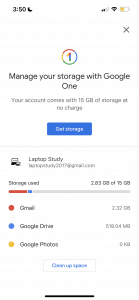The smartphone screen displays a user interface at 3:50 with a black crescent moon icon indicating Do Not Disturb mode, a half-full battery icon, and two bars for the cellular signal strength. Below this, on a white background, there's a large, multicolored number "1" inside a multicolored circle, representing the Google brand. Underneath in black text, it reads "Manage your storage with Google One," followed by a light gray text stating, "Your account comes with 15 GB of storage at no charge." 

A prominent bright blue button beneath this text says "Get storage" in white font. A pale gray horizontal line divides this section from the next. Under "Laptop study," indicated in black text with a laptop icon to its left, it shows storage information. The text "Storage used" in gray is followed by "2.83 GB of 75 GB" on the right, accompanied by a progress bar with a red line, a short bright blue line, and a long gray line, indicating the usage proportions.

The next section lists "Gmail" with a red dot, "Google Drive" with a blue dot, and "Google Photos" with a yellow dot. Beneath these labels, there is a white box outlined with a gray border containing the text "Clean up space" in bright blue.